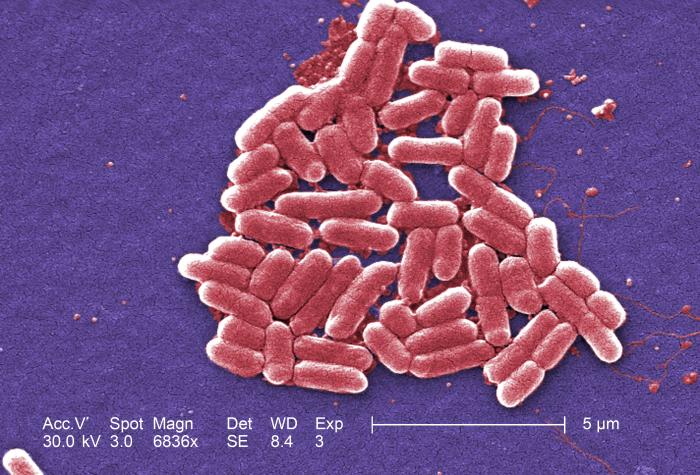Displayed is a detailed microscopic image of E. coli bacteria. Against a predominantly purple background, the pink-stained, long, and skinny, worm-like bacterial cells cluster together, their cylindrical bodies appearing fuzzy and slightly rounded at the ends. The image features various white text details at the bottom, including measurements and settings: "ACC.V 30.0 kV," "SPOT 3.0," "MAGN 6836X," "DET SE," "WD 8.4," and "EXP 3." A size scale indicating 5 micrometers allows for an understanding of the bacteria's dimensions.